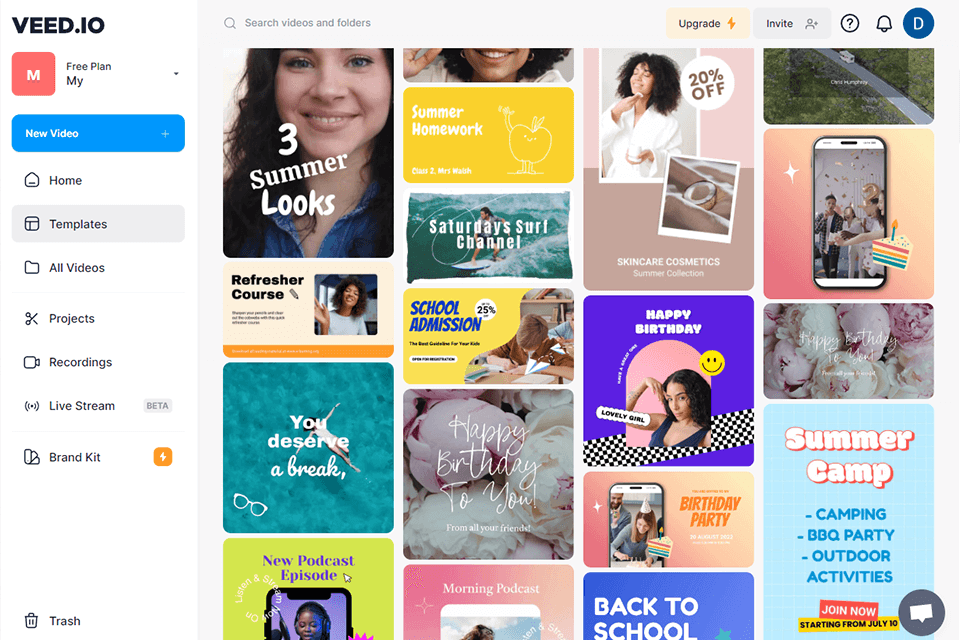## Detailed Caption for VEED.io Web Page

The web page displayed is for VEED.io, an online video editing platform. 

### Left Sidebar:
- **Logo and Plan Information**: At the top left corner, beneath the VEED.io logo, there's a box with a red background and a white letter "M" indicating the account type. Next to it, the text "Free Plan" is displayed, accompanied by a drop-down arrow.
- **New Video Button**: Below the plan information is a blue button labeled "New Video".
- **Navigation Tabs**: 
  - **Home**: Represented by a home icon.
  - **Templates**: Marked with a template icon.
  - **All Videos**: Depicted by a folder icon.
  - **Projects**: Shown with a scissors icon.
  - **Recordings**: Indicated by a camera icon.
  - **Live Stream**: Illustrated with a sound icon and labeled "Beta".
  - **Brand Kit**: Placed under the live stream option.
  - **Trash Can**: Located below the Brand Kit option.

### Top Right Bar:
- **Search Box**: Positioned at the top right.
- **Upgrade Button**: Located next to the search box.
- **Invite Button**: Situated beside the upgrade button.
- **Support and Notifications**: A question mark within a circle symbolizes support options, a notification bell icon for alerts, and a blue circular icon with the letter "D" indicates the user profile.

### Offers Section:
- Below the primary interface, there is a section listing various offers accompanied by images:
  - **Summer Homework**
  - **Three Summer Looks**
  - **Refresher Course**
  - **You Deserve a Break**
  - **New Podcast Episode**
  - **Saturday Surf Channel**
  - **School Admission**
  - **Happy Birthday to You**
  - **Morning Podcast**
  - **Back to School**
  - **Birthday Party**
  - **20% Off**
  - **Summer Camp**
  - **Camping**
  - **Barbecue Party**
  - **Outdoor Activities**
  - **Join Now**: With a note indicating the start date of July 10.

Each offer pairs with a relevant image, possibly as templates for various video projects.